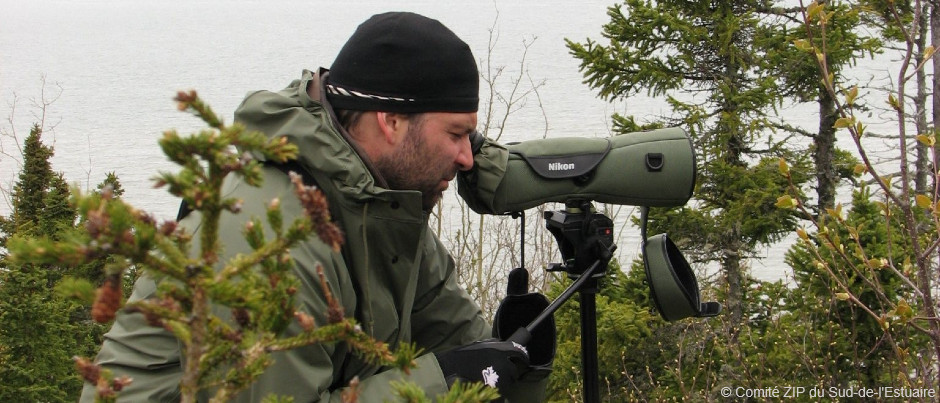In the image, a man is depicted in a woodland setting, closely examining a scene through a camera lens that sits atop a black pedestal tripod. He is dressed in an olive green jacket and a black knit cap, attempting to camouflage himself amidst the lush greenery surrounding him. The man, with a beard and mustache, is kneeling on the ground, his left hand gripping a bar extending from the camera setup, while his right hand is partially visible below the image frame. His left eye is closed as he peers through the viewfinder of the camera, which bears the brand name "Nikon" on its olive-covered body. The background is filled with evergreen trees and various foliage, and a hint of pale gray water can be seen further behind the trees, suggesting a natural, possibly forested, waterfront area. Additionally, another person can be faintly observed walking deeper into the background.